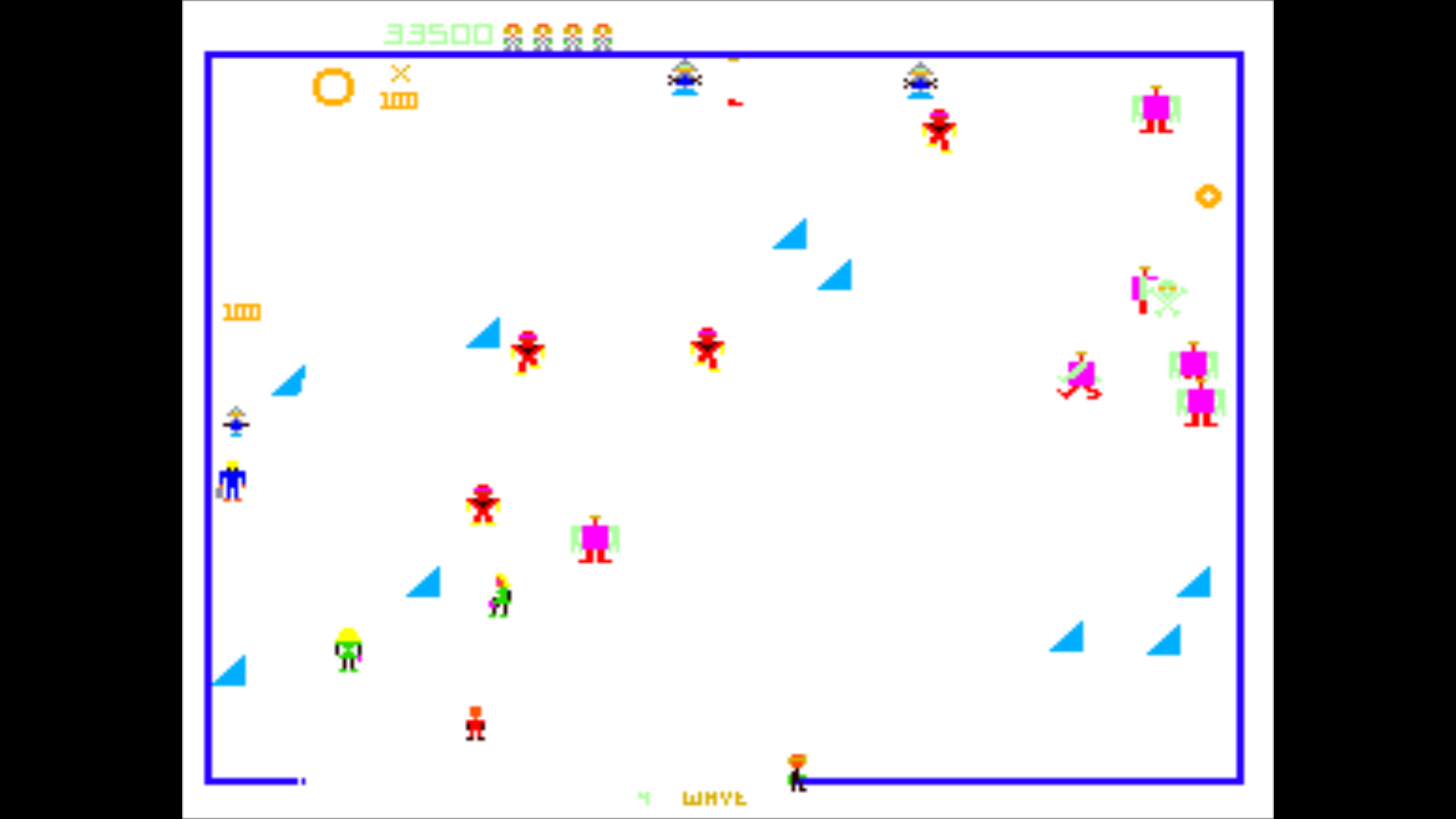This is a screenshot of a video game. The central part of the screen is dominated by a white rectangle, within which the game takes place. A dark blue outline encircles the edge of this white rectangle, resembling a football field. The player's score, displayed at the top left in green against the white background, is 33,500. To the right of the score are four little star indicators, representing character lives.

Scattered across the game field are various colorful objects: purple and green bots, red devil-like figures, blue right triangles, green bots, yellow circles, and two numbers that both indicate a thousand. At the very bottom of the white rectangle, the letters "WMVL" appear in yellow. This central game area is flanked by black bars on either side. The overall color palette of the game includes hues of purple, green, red, blue, and yellow, adding vibrancy to the white background.